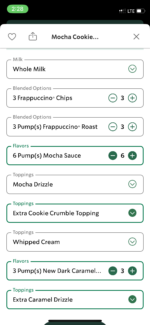A detailed order summary for a custom-blended beverage is displayed against a crisp white background. The central focal point is a vibrant green ordering interface highlighting the intricate customization of a 20-ounce mocha-flavored frappuccino. This specific order features a multitude of personalized options:

- **Base Ingredients**:
  - **Whole Milk**
  - **Ice**
  - **Frappuccino Chips**: 3 portions, adjustable with a green negative and plus sign.

- **Flavor Additions**:
  - **Frappuccino Roast**: 3 pumps (modifiable via green negative and plus signs).
  - **Mocha Sauce**: 6 pumps (modifiable with visible green adjustment signs).

- **Toppings**:
  - **Mocha Drizzle**
  - **Extra Cookie Crumble Topping**
  - **Whipped Cream**
  - **Extra Caramel Drizzle**

- **Additional Flavor**:
  - **New Dark Caramel Sauce**: 3 pumps (modifiable with green adjustment signs).

Visible at the top of the interface are essential icons:
- **Heart Icon**: Likely for favorites or saving the order.
- **Share Icon**: For sharing the custom order.

At the bottom of the display, there is a small black stand, providing a subtle contrast to the overall clean and vibrant aesthetic of the ordering screen. This meticulously detailed display ensures every ingredient and customization option is clear and adjustable, catering to the precise preferences of the customer.